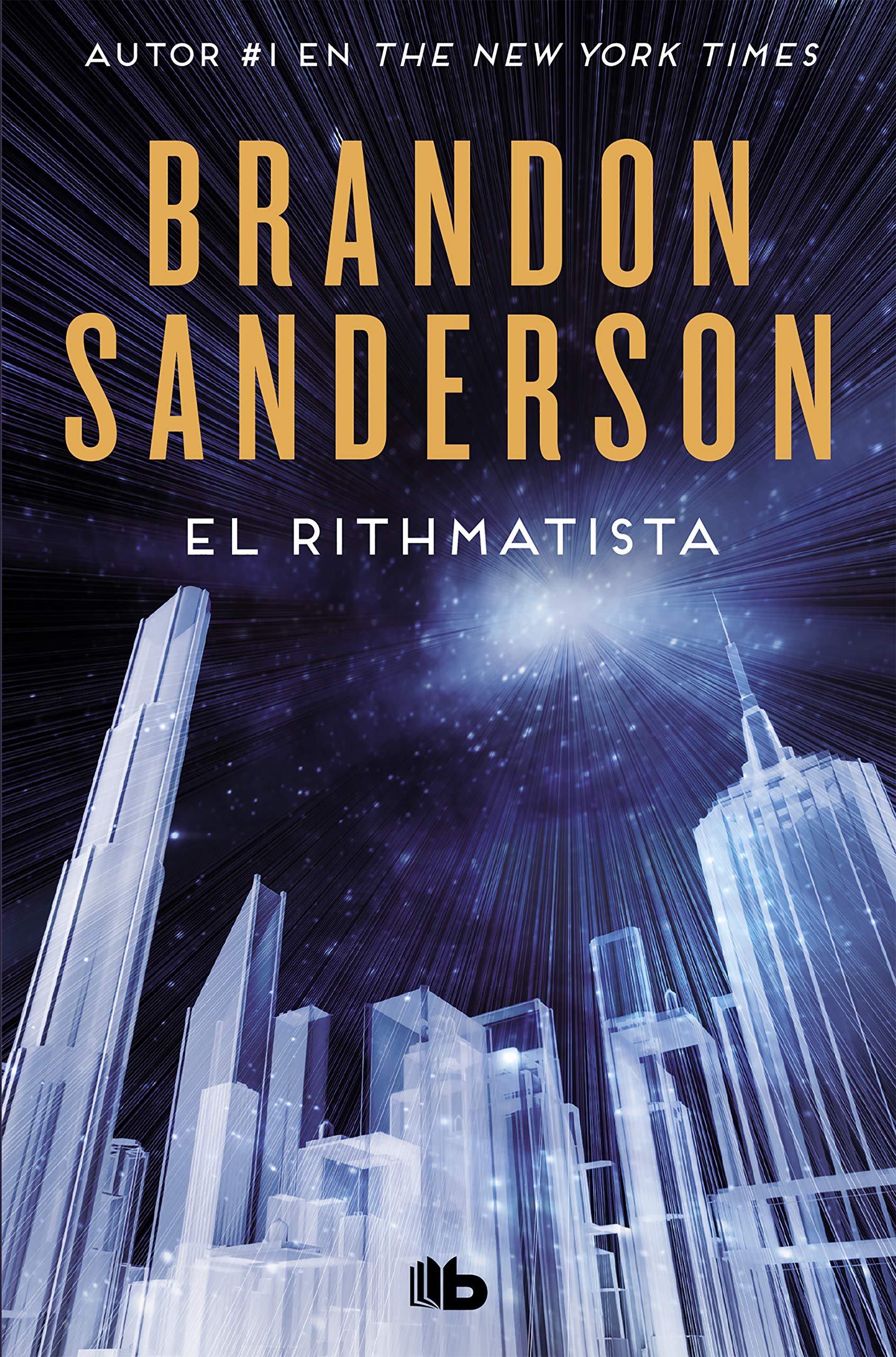The image features a book cover with the title prominently displayed. At the top, in white letters, it reads "Author Number One in the New York Times." Below this, in large, bold, yellowish-brown letters, is the name "Brandon Sanderson." Underneath his name, in smaller white letters, is the title "The Rithmatist." The bottom part of the cover showcases outlines of buildings that appear almost glass-like, giving the impression of a city skyline viewed from the ground looking up. The sky is a dark blue with a glowing white circle in the center, reminiscent of light shining down from the heavens. This celestial light illuminates the buildings, making them appear translucent and ethereal, as if they are bathed in a divine glow.